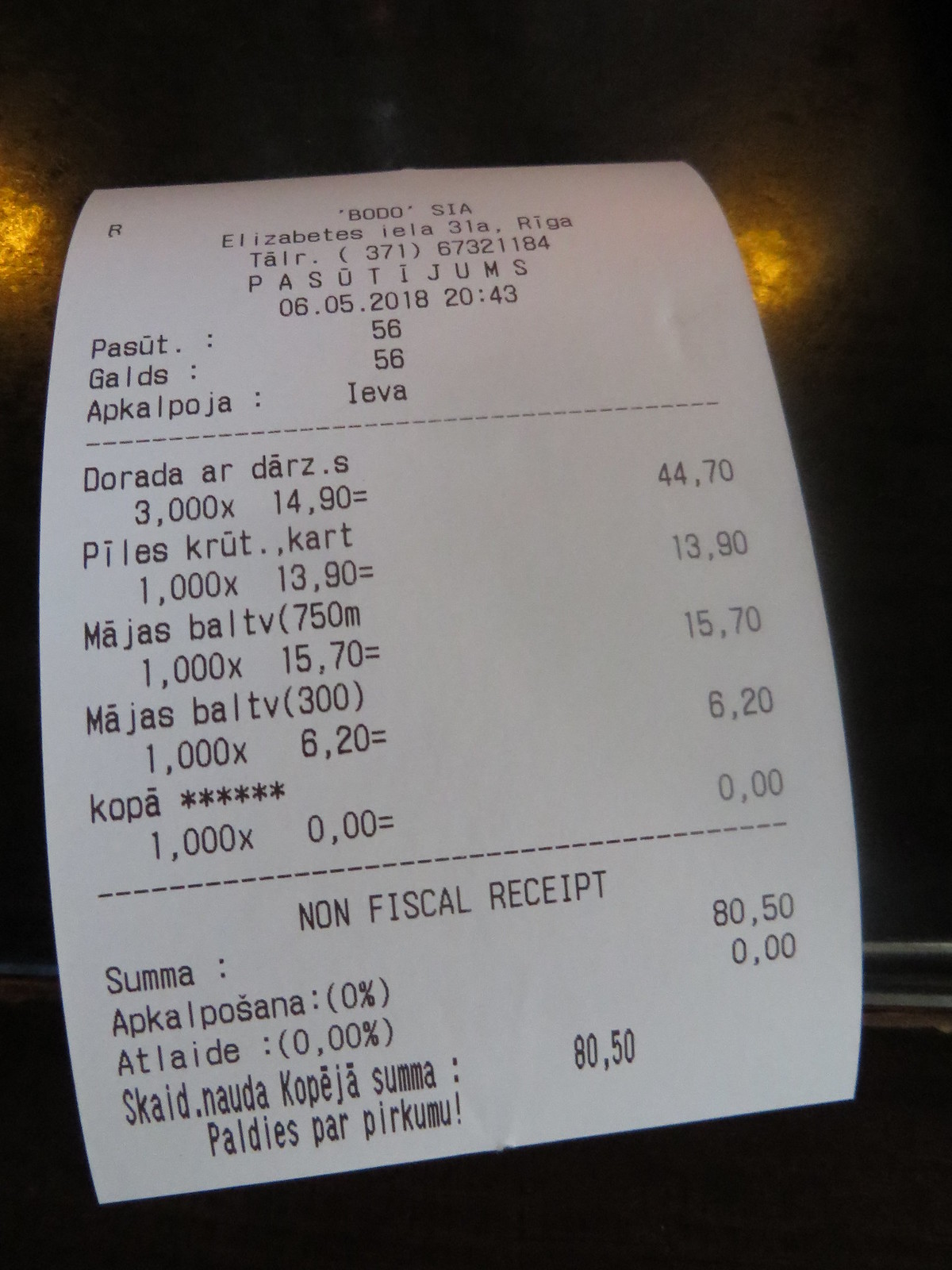The image showcases a small, slightly curved, white paper receipt placed on a dark brown or black surface. The receipt is illuminated by a light source, giving a slight reflection, including two yellowish dots from the light above. At the top, the teal slip has the text "Bordeaux, S.I.A," followed by names "Elisabeth, Iela, Triele, Riga, Tal" and a telephone number "371-673-21184." The receipt also includes the date "06-05-2018" and is written in a foreign language. The items listed are on the left, with their prices on the right: "Dorada Dars" priced at 44.70, "Peeled Crute Cart" at 13.90, "Madjaz Bulge" at 15.70 and another at 6.20, with "Coppa" priced at zero. The bottom of the receipt reads "Non-Fiscal Receipt" with a total amount of 80.50. Double white horizontal lines are visible at the bottom of the image, likely indicating the end of the receipt tape. The entire text on the receipt is printed in black.